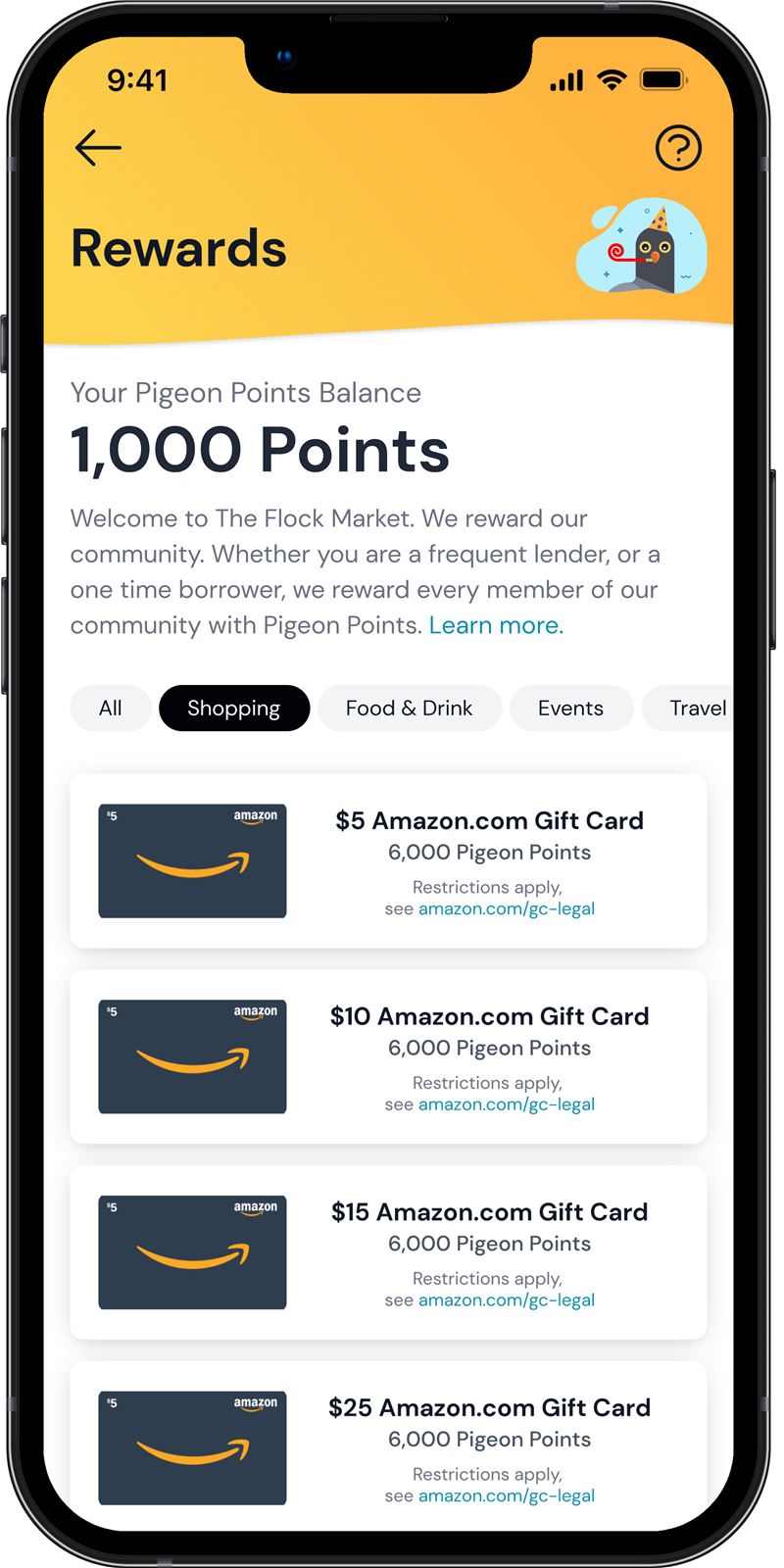**Descriptive Caption:**

This image captures a photograph of an iPhone screen, likely an iPhone 8 or newer. The screen displays a time of 9:41 AM and shows full cellular signal strength (4 bars), full Wi-Fi signal (3 bars), and a fully charged battery. The top section of the screen is divided into two parts: a smaller yellow section and a larger white section.

In the yellow section, a back arrow is visible in the top left corner, followed by the word "Rewards." On the right, there is a circular icon featuring a cartoon bird wearing a birthday hat with a question mark over it. Below this, it reads "Your Pigeon Points Balance" showing a balance of 1000 points. A subtitle beneath this states, "Welcome to the Flock Market. We reward our community whether you're a frequent lender or a one-time borrower. We reward every member of our community with pigeon points." A "Learn More" link appears to the right of this text.

The white section includes navigation tabs labeled "All," "Shopping," "Food & Drink," "Events," and "Travel," with "Shopping" being the currently selected tab. Below these tabs are four options for Amazon gift cards, each displaying an Amazon logo. 

- The first option: "$5 Amazon.com Gift Card" for 6000 pigeon points.
- The second option: "$10 Amazon.com Gift Card" for 6000 pigeon points.
- The third option: "$15 Amazon.com Gift Card" for 6000 pigeon points.
- The fourth option: "$25 Amazon.com Gift Card" for 6000 pigeon points.

Each gift card option includes the note "Restrictions apply" and a link to Amazon.